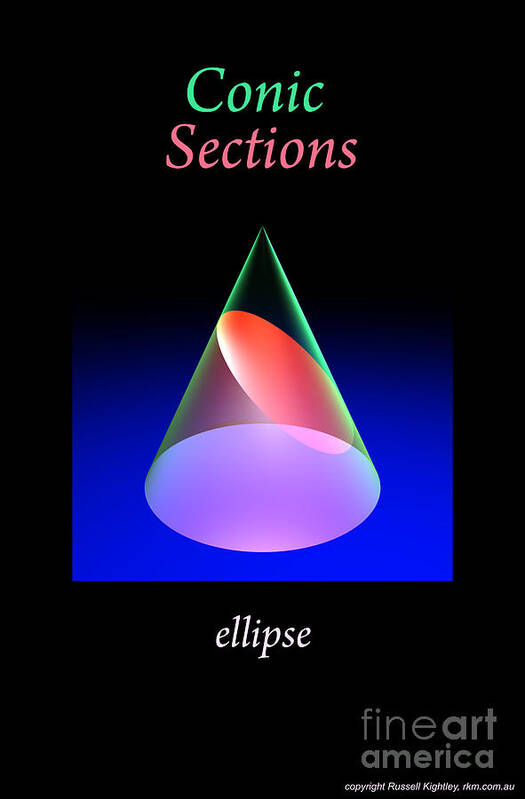This image features a poster set against a black background, with a prominent blue section in the middle. At the top of this blue section, "Conic" is written in green text with a capital 'C', followed by lowercase letters. Beneath this, the word "Sections" is displayed in pink text. The central focus is an upside-down cone angled upwards, making its interior visible, accented with a green border. Inside the cone, there's a prominent reddish oval shape, while the top face exhibits a purple hue. At the bottom, the word "Ellipse" is shown in white text. In the bottom right-hand corner, the poster notes "Fine Art America" in gray text, with "Fine" in a slightly thinner font compared to "Art" and "America". Below this, it reads "copyright Russell Knightley" and "RKM.com.au".